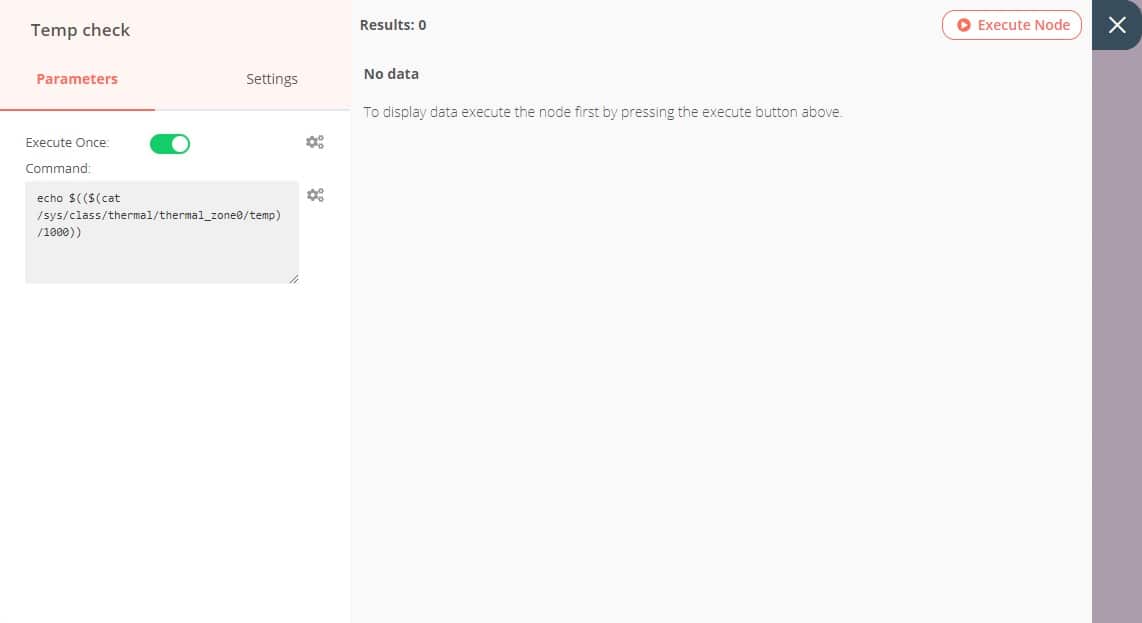The image shows a user interface for system configuration and monitoring, specifically for managing thermal parameters. The interface features options like 'Temp', 'Parameter Settings', and 'Execute Once'. Users can toggle commands such as 'Echo' and 'Cat', and navigate through system classes like 'Thermal' and 'Thermal Zone'. The displayed parameters include 'Temp' with a value of 1000. Currently, results are showing 'zero' with no available data. To display the necessary data, the user must first press the 'Execute' button located above the node. An 'X' icon is present in the top right corner for closing the interface.